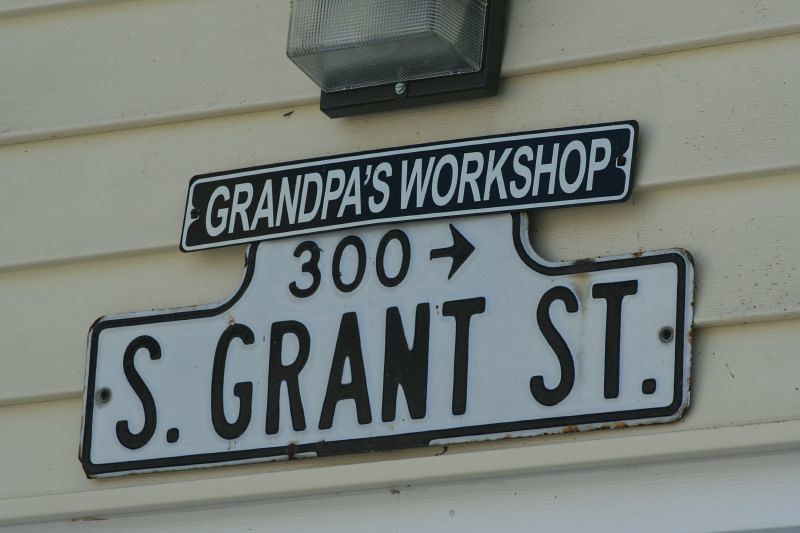This image captures an up-close view of a metal sign mounted on the pale yellow siding of a building. The focal point is a rectangular black sign with white lettering that prominently reads "Grandpa's Workshop." Directly below this is another larger white sign with black text reading "300" followed by a right-pointing arrow and "S. Grant St." Above these signs, there is an outdoor light fixture featuring a crystal-patterned cover, providing illumination. The overall composition suggests that this sign, reminiscent of a street sign, designates a specific location, potentially a workshop or business, integrated into the building's exterior decor.